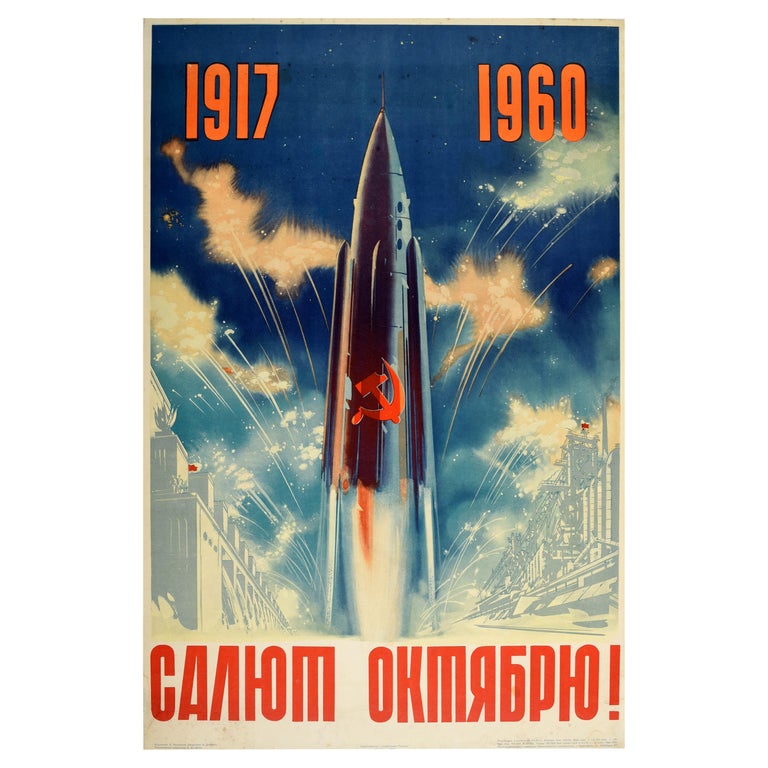This vintage poster, reminiscent of the Russian space race era, features a prominent Soviet rocket ascending into a deep blue, star-studded sky. The poster's border is a yellowish hue, framing the central image strikingly. At the top, the year "1917" appears in orange on the left, while "1960" is displayed on the right. The rocket, predominantly dark gray or black, bears the iconic red hammer and sickle symbol of the Soviet Union on its upper section. The rocket's body transitions to silver with a splash of orange, suggesting the energy of liftoff. White streaks emanate from the rocket's base, enhancing the sense of dynamic motion. Surrounding the rocket, wisps of white clouds and brilliant stars dot the sky. Flanking the scene are brick buildings that evoke an official aura, possibly hinting at the Kremlin. The bottom of the poster showcases a bold red Russian inscription with an exclamation point, emphasizing the dramatic and celebratory tone of the image. The overall composition captures the historical significance and ambitious spirit of the Soviet space endeavors.